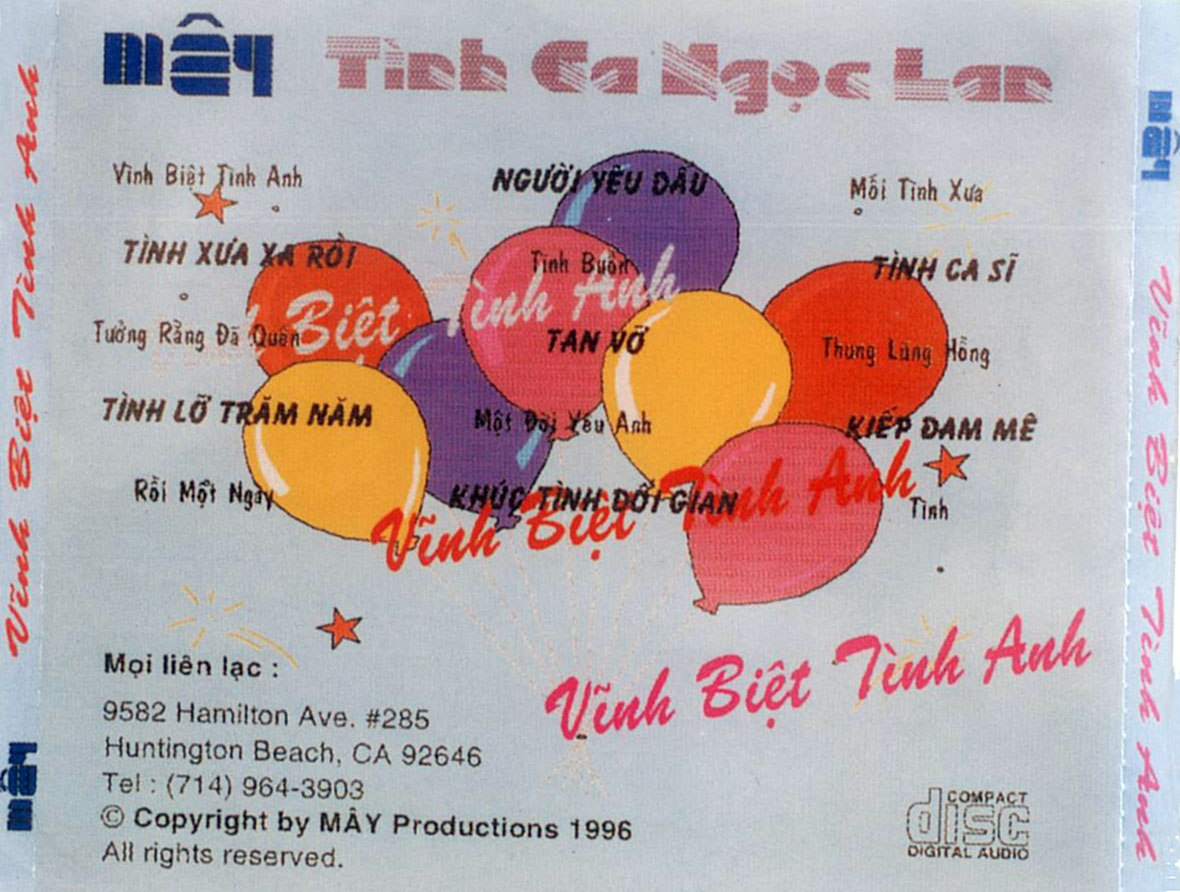This image features a compact disc cover set against a white background with intricate lettering, predominantly in Vietnamese. The upper portion of the cover displays a mix of bold, thick blue, pink, and red text, possibly indicating the title "Vinh Biet Tinh An." Surrounding the text are illustrated balloons in a recurring pattern of yellow, red, purple, and a darker reddish-pink, with several orange stars interspersed among them. Overlaying the balloons, the titles of different songs are written in various colorful fonts. Along both the left and right vertical edges of the cover, there are vertical lines of text in blue, red, and pink, also in Vietnamese. Nestled in the lower right corner, the familiar compact disc digital audio logo appears, while the lower left corner provides detailed contact information: 9582 Hamilton Avenue, Number 285, Huntington Beach, California 92646, along with a telephone number. Additionally, the cover includes a copyright notice, "Copyright by May Productions 1996, All rights reserved."